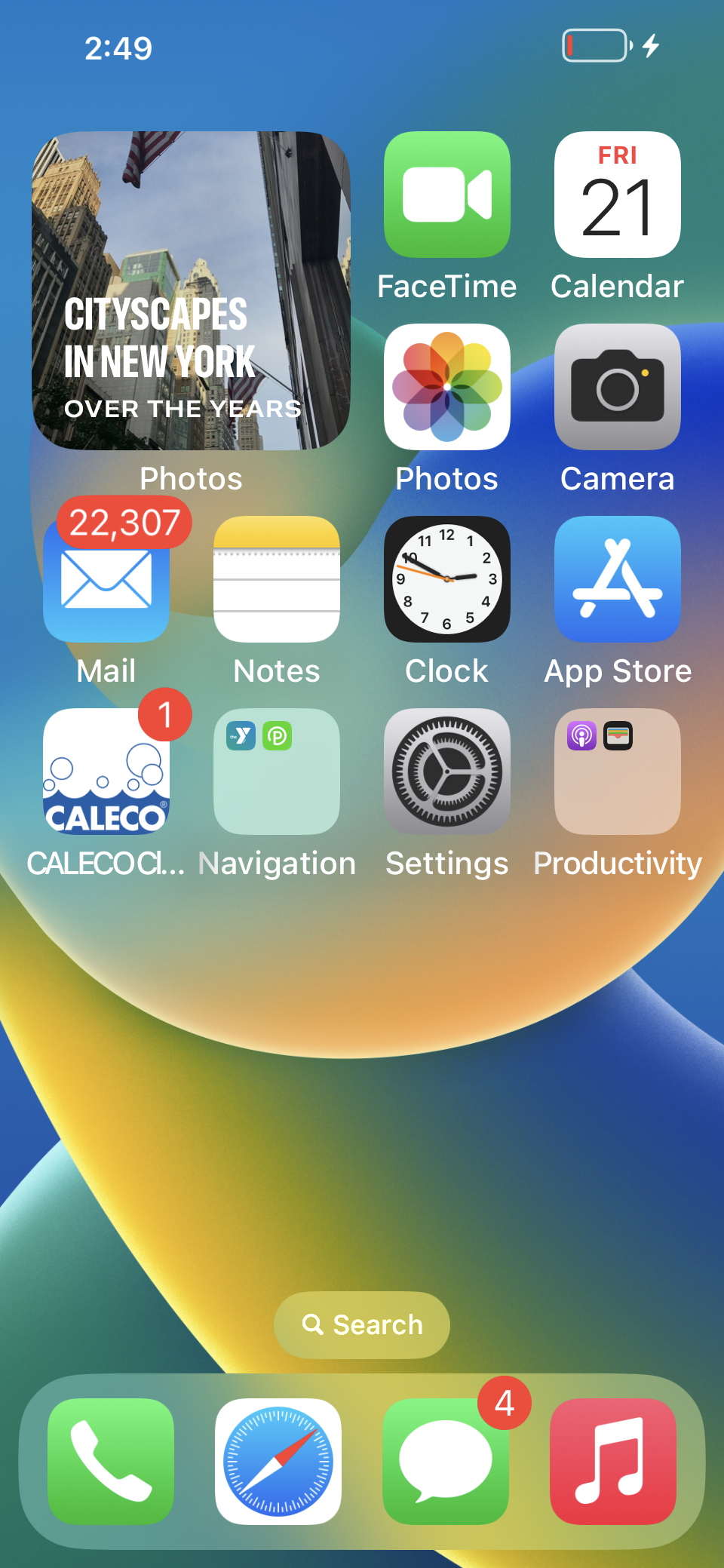The image displays the screen of an iPhone, showcasing a variety of apps. What makes this phone screen particularly intriguing is the background image of the cityscape of New York, which is tied to a large application labeled "Cityscapes in New York Over the Years." The background image captures an upward-looking perspective from the ground level towards towering buildings, framed against a bright sky.

The screen includes several standard iPhone apps arranged in a familiar layout: FaceTime, Calendar, Photos, Camera, Mail (which has over 22,000 unread messages), Notes, Clock, App Store, Calculator, and Navigation. Additionally, the settings and productivity folders are clearly visible.

At the bottom of the screen, there's a search bar and a dock featuring the most recently used apps, including the Phone, Compass, and Messaging app (indicating four unread messages). Additionally, there is an icon featuring a music note, possibly representing Apple Music.